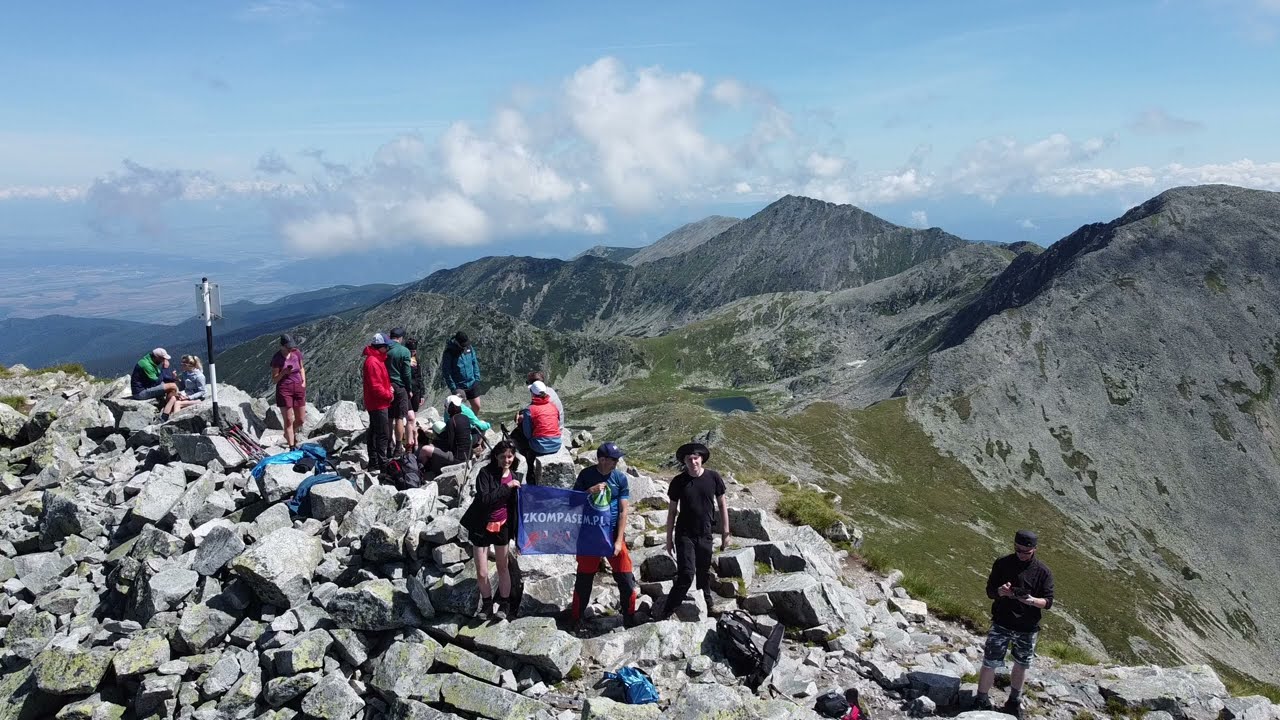This photograph captures a group of roughly a dozen to twenty people climbing a rocky mountaintop, characterized by large gray rocks with patches of lime green moss. Two central figures face the camera, holding a translucent blue flag inscribed in white with "ZKOMPASEM.PL." The climbers, dressed in various colors such as red, blue, orange, black, and white, appear relaxed and casual, possibly part of a hiking group or an organized outing like a school field trip or Boy Scouts. The backdrop reveals a darker mountain range dotted with dark green moss, with peaks reaching towards a light blue sky with fluffy white clouds. Images of other hikers are visible in the background, possibly hinting at a busy and shared outdoor adventure.